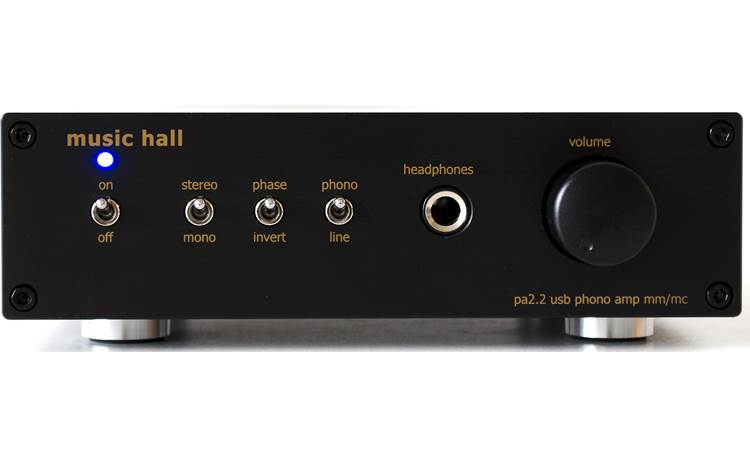This image features a detailed close-up of a professional black preamplifier, ideal for a musical venue or auditorium, though it may also be used residentially. The preamp prominently displays a label on the bottom right corner that reads "PA 2.2 USB Phono Amp MM/MC." On the front panel, from left to right, there are several controls: the top-left corner features a small blue LED light indicating power status. Directly beneath it is an on-off switch labeled "On" at the top and "Off" at the bottom. Next is a switch for selecting between "Stereo" and "Mono" modes, followed by a switch for "Phase" (top) and "Invert" (bottom) functions. The fourth switch toggles between "Phono" (top) and "Line" (bottom) inputs. Adjacent to these switches is a headphone jack labeled "Headphones," and to the far right, there is a large volume knob marked "Volume." The preamp is set against a white background, emphasizing its sleek, functional design.